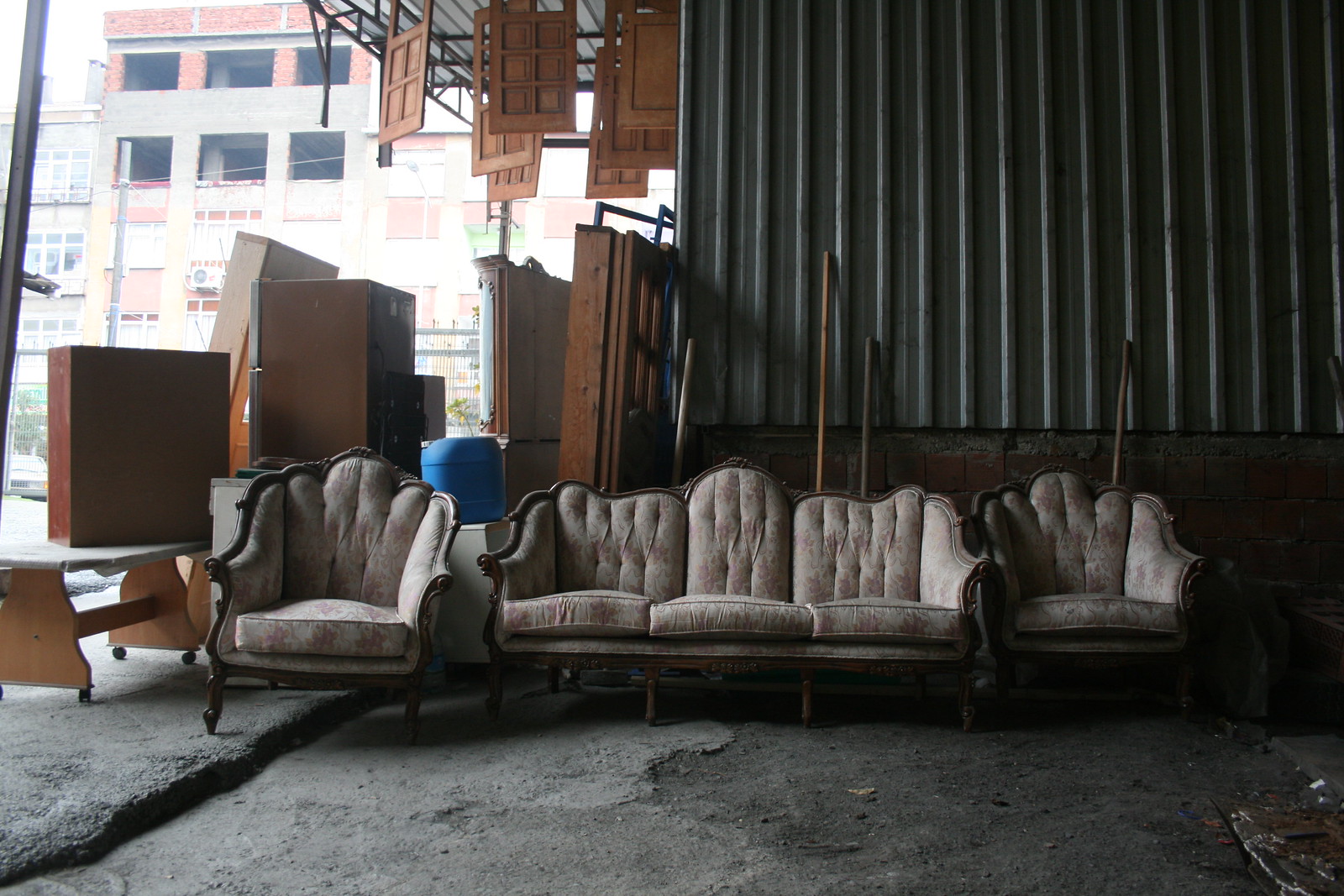This image depicts an outdoor furniture repair shop with a rustic, industrial aesthetic. Dominating the scene is a lineup of matching antique furniture, comprising a three-seater couch flanked by two armchairs. These pieces feature intricate dark brown wood framing and off-white upholstery adorned with a pink floral pattern. The seating arrangement rests on a rough, dirty concrete floor bordered by a corrugated metal wall on the right. The upholstery appears worn and in need of repair, with visible rips. To the left, the setting extends outdoors where additional furniture, including tall shelves and a brown refrigerator, is visible. Suspended from the roof of this metal shed are various doors or window shutters, adding to the eclectic collection. In the background, a stark, industrial brick building adds to the gritty charm of the setting.